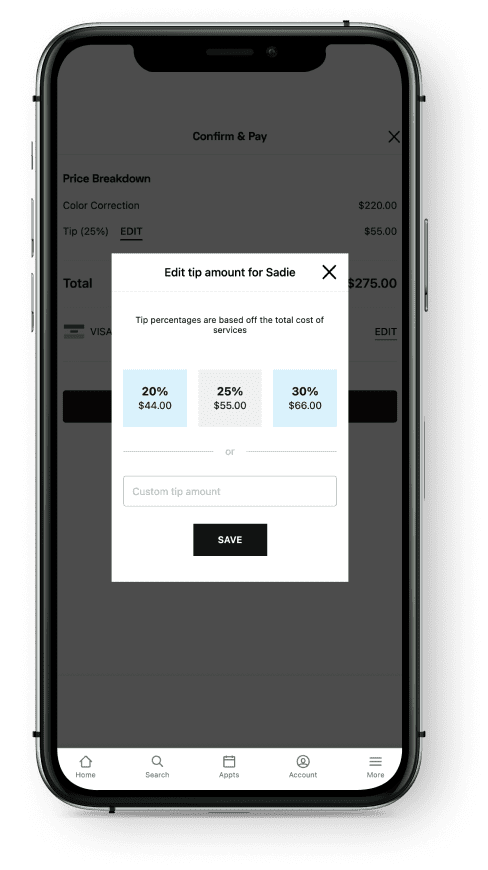A black-outlined smartphone screen is depicted in the photo. The main interactive section displays the heading "Confirm and Pay" in a grayed-out font. Below that, the "Price Breakdown" includes a service labeled as "Color Correction" priced at $220, and a tip amount calculated at 25%, which is $55. 

An overlay window titled "Edit Tip Amount for Sadie" is also visible. This pop-up explains that "Tip percentages are based off of the total cost of services." It presents three tip percentage options: 20% for $44 (highlighted in blue), 25% for $55 (centered), and 30% for $66. A gray separator below these options includes the word "or," followed by a "Custom Tip Amount" box where users can input a different tip value. Beneath this, a black "Save" button is clearly visible.

The remainder of the screen is white with a faint gray background. At the very bottom of the screen, a navigation bar includes icons labeled "Home," "Search," "Apps," "Account," and "More."